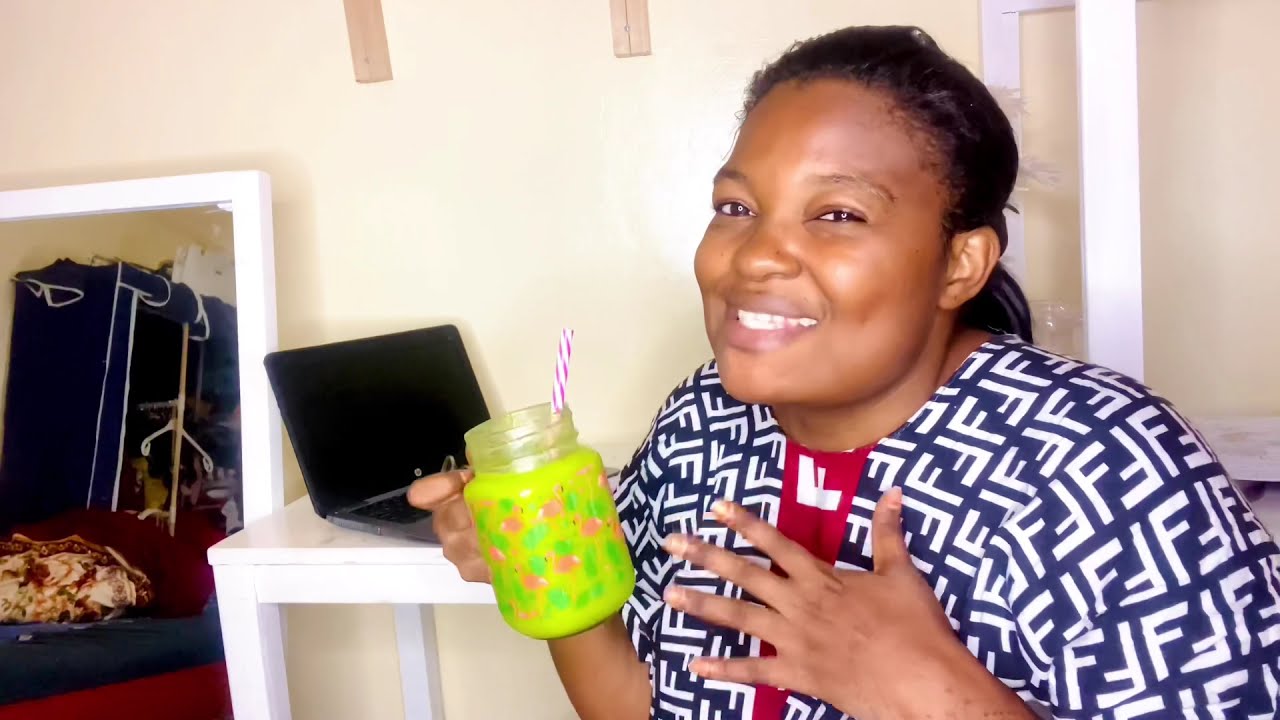The photograph captures a joyful black woman standing to the right, holding a jar with green liquid and a pink and white straw in her right hand, while her left hand is extended in front of her chest, displaying her fingers and fingernails. She is smiling broadly, her face turned slightly to the side but looking straight into the camera. The woman is dressed in a blue shirt adorned with a pattern that includes white and a bit of red. To the left of the woman on a white table is an open but inactive laptop, and further left, there's a mirror with white borders that appears to reflect a wardrobe. A white bottle is visible to the right of the woman. The background features a cream-colored wall with two brown rectangles near the ceiling, along with a grey country-style shelf positioned beside the woman.